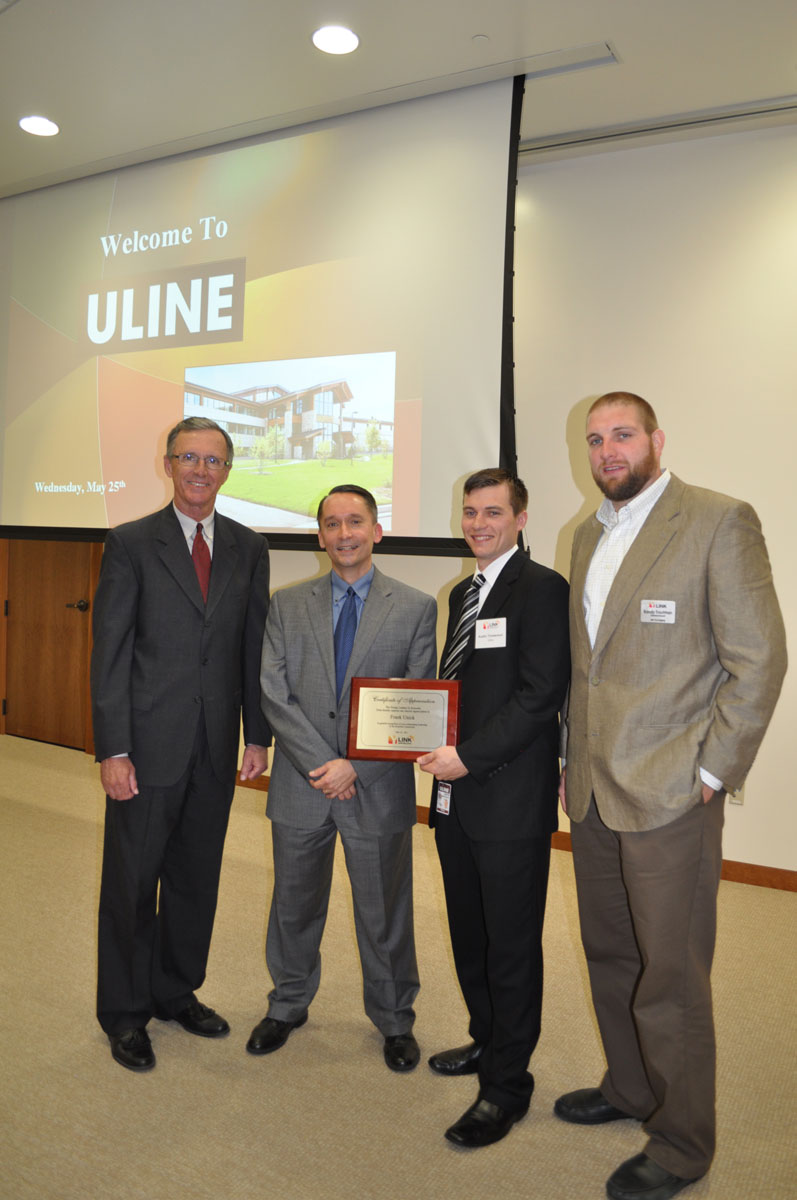In this detailed indoor photograph, four well-dressed men are standing in a line on tan-colored carpeting, facing the camera. Behind them, a projector screen displays the message "Welcome to Uline" with an image of a building and the date, "Wednesday, May 29th." The men are wearing suits in various colors: a black suit with a red tie and glasses on the roughly 60-year-old man on the left; a gray suit with a blue tie on the man next to him, who has his arms crossed; a black suit with a visible name tag on the third man, who is holding an award with a maroon background; and a brownish suit with a beard and white undershirt on the man furthest to the right, who is the tallest. They all have black shoes and are positioned at different angles to the camera but are all looking straight ahead. The lighting and environment suggest the photo was taken indoors, although it is unclear whether it was daytime or nighttime.